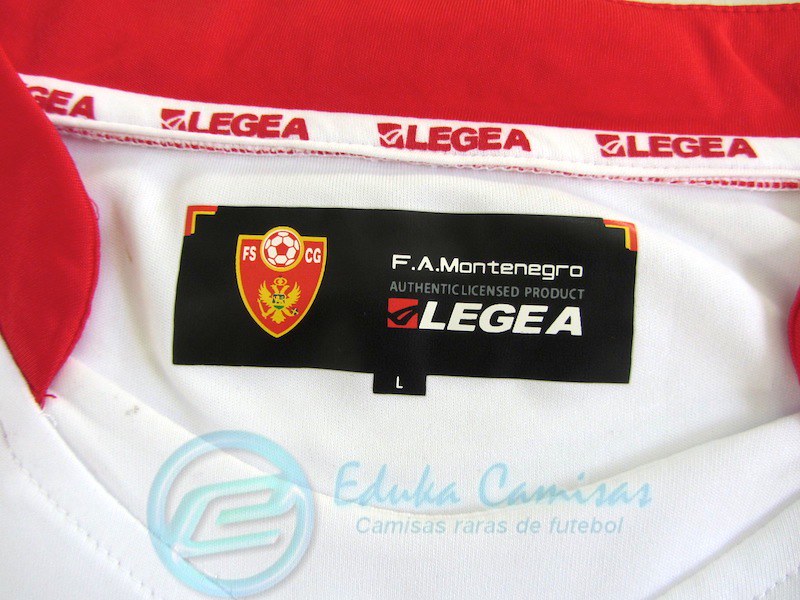This image displays a close-up of the label on a white soccer jersey with red accents, specifically focusing on the collar area. The jersey features a red collar and a white band inside the collar with the logo "Legea" spelled out in red letters, accompanied by a red symbol on its left side. 

The tag inside the jersey is a horizontally oriented black rectangle with red and yellow outlines at the top corners. Prominently on the left side of the tag is a shield logo with "FSCG" written in the top sections of the shield, featuring a football at the top and detailed imagery including a bird with a sword and a weapon at the bottom. On the right side of the tag, it states "FA Montenegro, Authentic Licensed Product, Legea." 

The jersey is identified as a size large, indicated by the letter "L" on the tag. Below this, there is a watermark featuring a light blue "E" within a circle, along with the text "Educa Camisas, Camisas Juarez de Futbol," suggesting it might be in Spanish.